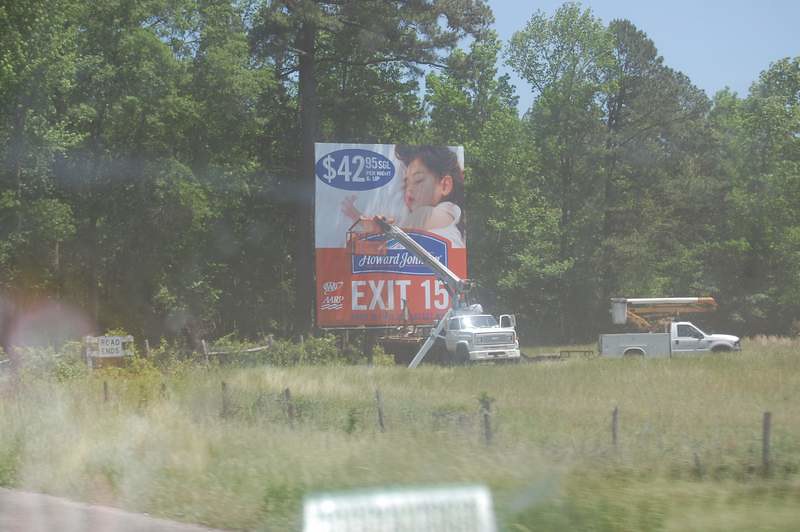The image depicts a lush, green grass field with a wire fence running diagonally from the bottom right corner to the left. At the corner of the fence, a white banner is displayed, stating "Routine Road Ends" in black letters. The central focus of the photograph is on two white construction trucks amid a sprawling outdoor setting that appears to be either a farm or a forest area, under a clear blue sky.

The primary truck in the center, with its left door open, features a black trailer and an extended crane arm reaching upwards towards a large billboard. The billboard, which seems to be a hotel advertisement for Howard Johnson, is detailed and colorful. On the top left of the advertisement, it displays "$42.95" in white text against a blue oval background. Just to the right, a sleeping child is depicted on white bedsheets. The banner further down features "Howard Johnson" in white, set within a blue square and is highlighted by a red border emphasizing "EXIT 15".

To the right of the central truck is another white vehicle with a yellow crane, which is not extended. Surrounding the trucks are very tall trees with varying shades of green leaves, contributing to the serene and expansive feel of the scene. In the background, the tops of these trees stand out against the blue sky. There are also elements such as the "Road Closed" sign, which appears discarded among the woods to the left, and additional white objects scattered towards the bottom of the image, adding to the realistic outdoor working environment.